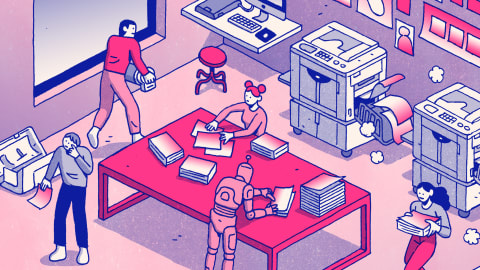The image is a cartoonish illustration depicting a collaborative scene in a print shop. In a pink and lavender color palette, the characters and settings are illustrated with simple, comic-like features. The scene prominently features four human characters—two women and two men—and one pink robot, all working together amidst bustling activity. 

In the foreground, a woman with bright pink hair styled in buns above her ears is seen stacking papers on a pink table alongside the robot, which is sorting sheets. Another woman is carrying stacks of paper from the printers in the background, which are actively spitting out pink sheets of paper. One man, dressed in blue pants, holds a sheet of paper in his right hand while touching his face with his left. Another man with dark pink pants and a matching shirt is carrying a cylindrical object and walking towards a desktop computer set up on a stool in the corner. Despite the presence of a window, there is no visible scene outside. Scattered balls of paper clutter the floor, enhancing the busy atmosphere.